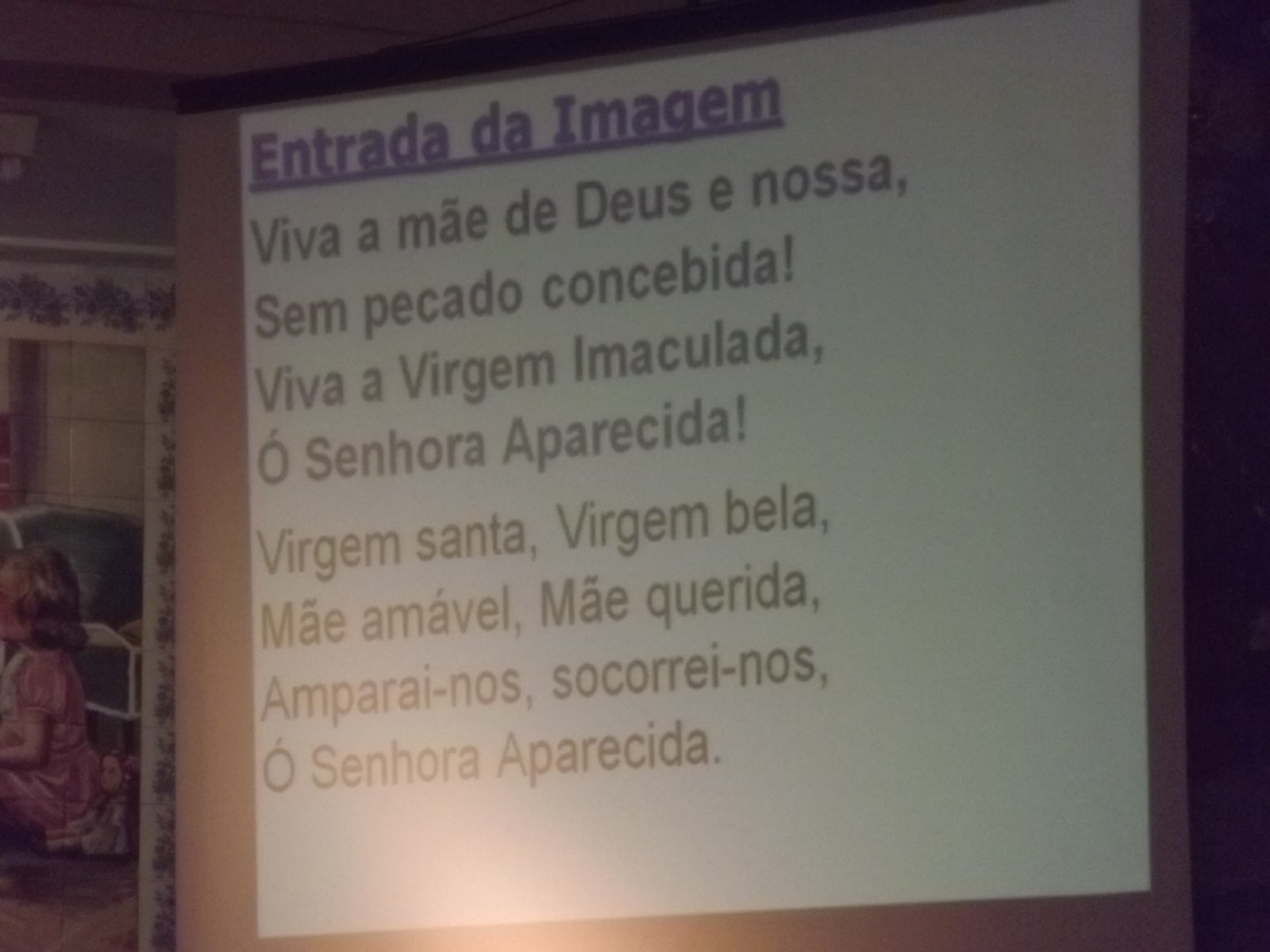The image depicts a slightly blurry and dark picture of a presentation slide projected on a white screen, possibly in a small church. The background of the slide is white, and it contains only text without any clip art or images. At the top, the title "Entrada da Imagem" is written in bold, purple ink and underlined. Below the title, the rest of the text, which appears to be a poem or prayer, is written in black ink. The text is divided into stanzas with punctuation at the end of each line, and it is in Portuguese. The words of the poem or prayer include phrases like "viva a mae de Deus e nossa," "sem pacado concebida," "virgem imaculada," "virgem santa," "virgem belas," "mae mamável," "mae querida," "amparainos," "socorreinos," and "o senhora aparecida." In the background, behind the projector, there is a glimpse of a painting on the wall showing a little girl in a pink dress sitting on the floor, framed by a white border adorned with vine details. The overall setting suggests a reverent atmosphere, possibly during a religious service.